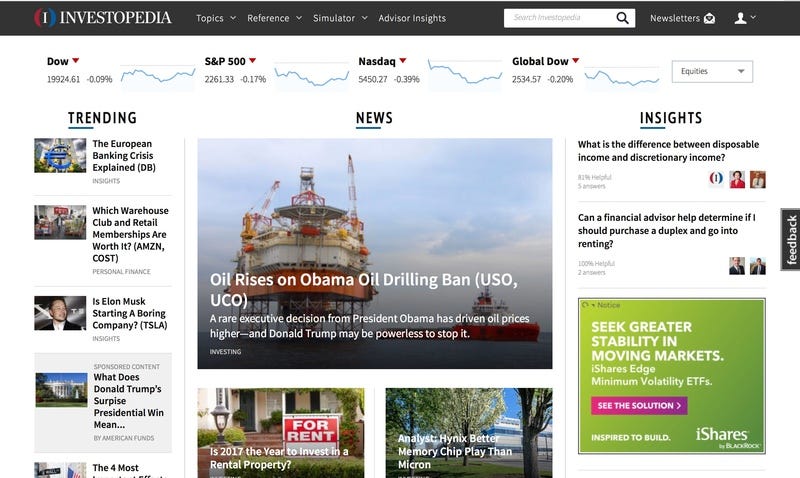Here’s a cleaner and more detailed caption for the image described:

---

The image displays a webpage with a white background featuring the Investopedia logo. Centered prominently is a black box with an eye symbol, framed by blue and red lines, and accompanied by the labels Topics, Reference, Simulator, Advisor, and Insights. Adjacent to these labels, there is a search box and icons for newsletters and account management.

Scrolling down, a section is dedicated to the stock market with updates on the Dow Jones, trending topics, and articles such as "The European Banking Crisis Explained," "Which Warehouse Club and Retail Memberships Are Worth It?", and "Is Elon Musk Starting a Boring Company?" A blue highlighted box poses the question, "What Does Donald Trump's Surprise Presidential Win Mean?" though part of this section is cut off.

Beneath a dividing line, there is a larger section with a significant headline, "Oil Rises on Obama's Oil Drilling Ban," followed by stock symbols USO and UCO. The financial indices displayed include S&P 500, NASDAQ, Global Dow, and an equities box. 

Further down, two smaller images are titled "Is 2017 the Year to Invest in Rental Property?" and "An Analyst Panics: Better Memory of Clip Play than Micron." Another dividing line separates these entries from content on the right.

The "Insights" section is underlined with a green bar, featuring an article "What is the Difference Between Disposable Income and Discretionary Income?" Below this, two smaller images explore whether a financial advisor can help decide if purchasing and renting a duplex is advisable.

To the right, there is a vertical black box for feedback. A green box encourages seeking greater stability in moving markets with "Shares Edge Minimum Volatility ETFs," accompanied by a purple button labeled "See the Solution." An iShares promotional caption concludes the section with "Inspired to Build."

---

This caption encapsulates the elements and layout of the webpage, providing a detailed description of the visual and textual content present in the image.